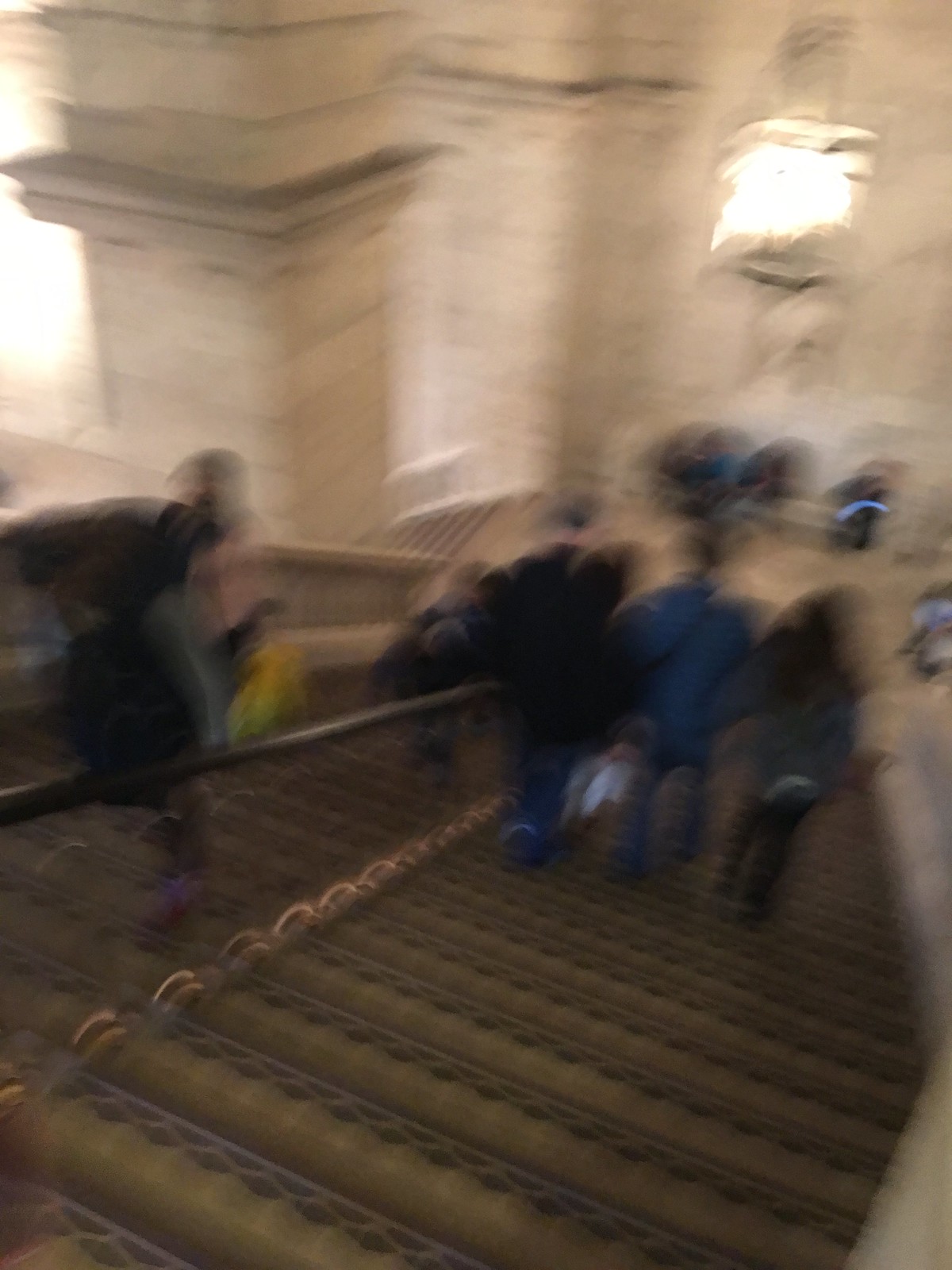An out-of-focus image captures the scene of a group of people descending a wide staircase. The background is largely indistinct due to the blur, but white walls and a prominent stone pillar on the left-hand side are faintly discernible. At the center of the image, three individuals with dark hair and dressed in dark clothing can be seen making their way down the stairs. To their left, additional figures are visible, though their direction is unclear due to the blurred quality of the photo. Natural daylight streams in from what appears to be a large window on the left side, illuminating the scene with a soft, diffused light.